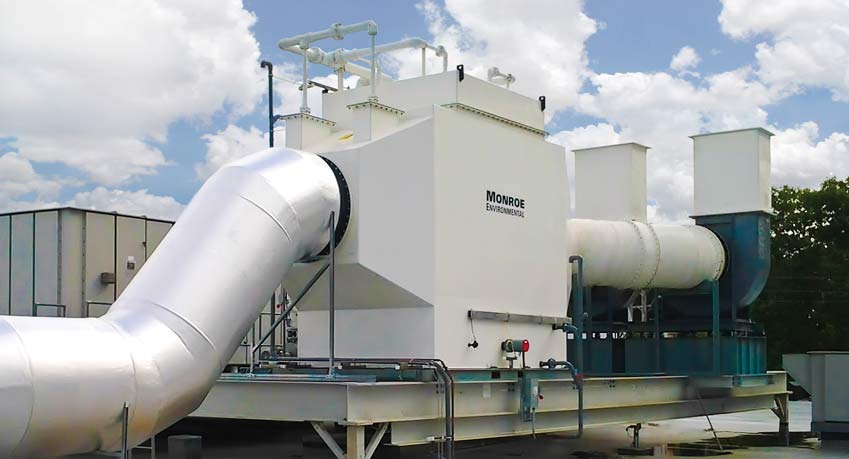In an outdoor factory setting, a prominent piece of machinery dominates the scene against a backdrop of blue sky and large white puffy clouds. The machinery, comparable in size to a mobile home, features a large white rectangular unit labeled "Monroe Environmental" in black lettering. Atop this unit is complex piping, and extending from its center is a substantial silver aluminum tube that curves down before leveling out. Another significant tube, white in color, protrudes from the left side, connecting to a green curved metal area capped with a white rectangular structure resembling smokestacks, though no smoke is visible. Behind the machinery, there is a metal building with aluminum siding and a flat roof. On the right-hand side of the image, green trees are visible, adding to the outdoor industrial atmosphere.